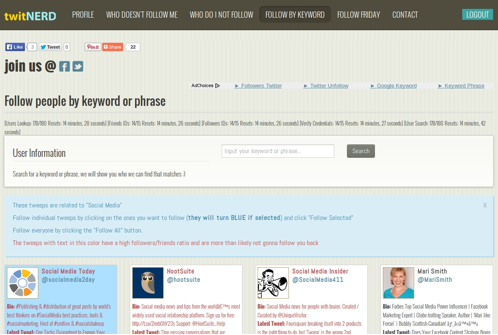This screenshot features a tech website called "Twit Nerd." The website's name is prominently displayed at the top left in colorful text, with "Twit" in yellow and "Nerd" in baby blue. The logo is situated on a light brown banner that spans the top section of the page.

Directly below the banner, there's a row of navigation tabs featuring options such as "Profile," "Who Doesn't Follow Me," "Who Do I Not Follow," "Follow by Keyword," "Follow Friday," and "Contact," all presented in white text. 

Beneath the logo, users find social media interaction buttons labeled "Like," "Tweet," "Pin," and "Share," allowing easy sharing across various platforms. Below these options, there is a call to action: "Join us at Facebook, Twitter," accompanied by the respective logos of these social media sites.

Additionally, there is a prominent text section inviting users to "Follow key people by keyword or phrase," written in black. Within this area, a user information bar prompts visitors to "Search for a keyword or phrase," promising to showcase matching profiles based on the input.

Although the exact nature of this website is unclear, it appears to be a tool designed for social media research, likely focusing on finding and following users across Twitter and Facebook based on specified keywords or phrases.